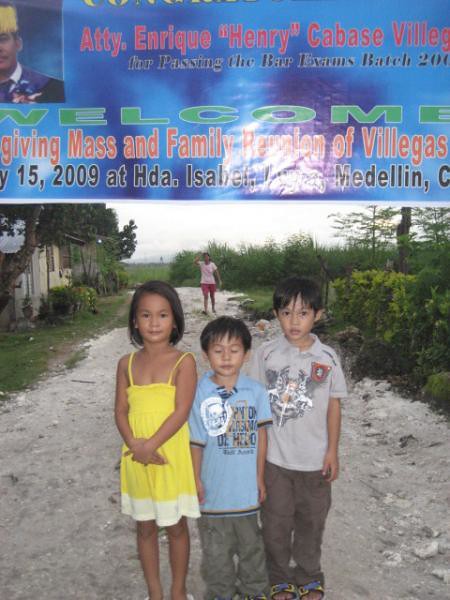In a rural, countryside setting on a dirt road flanked by lush greenery, three children, appearing to be of Filipino descent, pose for the camera. To the left stands a young girl in a vibrant yellow sundress, while beside her, two boys wear shirts with graphics—one in blue and the other in gray. Notably, the boy in the blue shirt stands in the middle with his eyes closed. To the left in the background, there's a rundown house adding a rustic charm to the scene. Further down the road, an indistinct figure in a white shirt and red shorts walks towards the children, set against a cloudy sky that casts a muted light over the charming, weathered landscape.